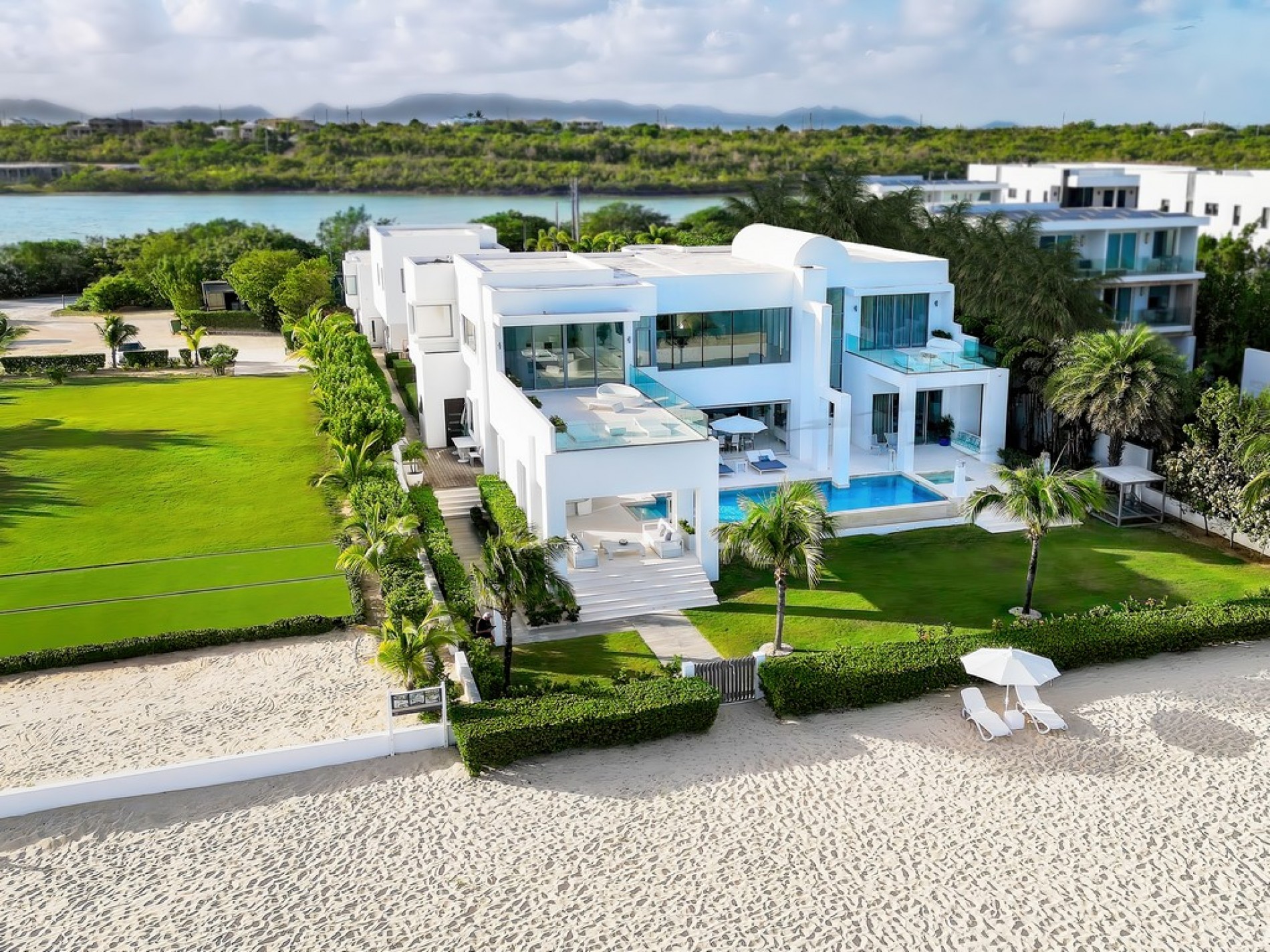This is an aerial photograph, possibly taken by a drone, of a luxurious white beach house that exudes Miami vibes. The house features a modern, blocky cube design with floor-to-ceiling windows in nearly every room. In front of the house, there's a shimmering swimming pool bordered by lounge chairs and a well-maintained lawn. Beyond the lawn, a hedge separates the property from a sandy beach that spills into a body of water. The picturesque scene includes palm trees scattered throughout the yard, enhancing the tropical ambiance. Behind the house lies another multi-story structure, hinting at a neighboring river or lagoon. The photograph captures a serene moment with the sun low in the sky, casting long shadows over the flat terrain. The setting is tranquil and completely devoid of people, presenting an idyllic yet private coastal retreat. Clouds hover gently above, framing a perfect seaside escape that could very likely be nestled in Florida, possibly Miami.